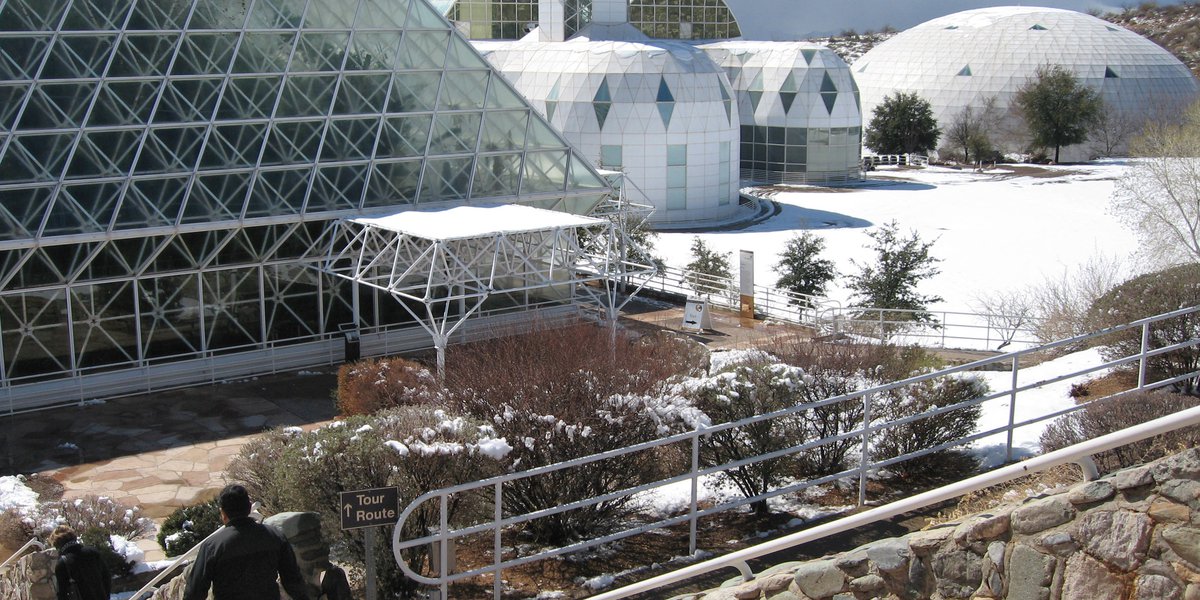This photograph captures a striking scene featuring a distinctive architectural exhibit, blanketed in an unexpected layer of snow. The focal point is a large, white geodesic dome in the background, characterized by triangular geometric frames. Adjacent to it are several dome-like and bunker-style structures, including a notable glass building with triangular intersections forming an elaborate frame. In the foreground, a gray stone wall and a sign indicating the "tour route" can be seen, directing visitors toward the buildings. Although it's unusual to see snow in this locale, which is believed to be in Arizona, the presence of snow adds a unique element to the landscape. Visitors are visible walking towards the exhibit, enhancing the sense of scale and the human interaction with this fascinating, enclosed ecological environment.